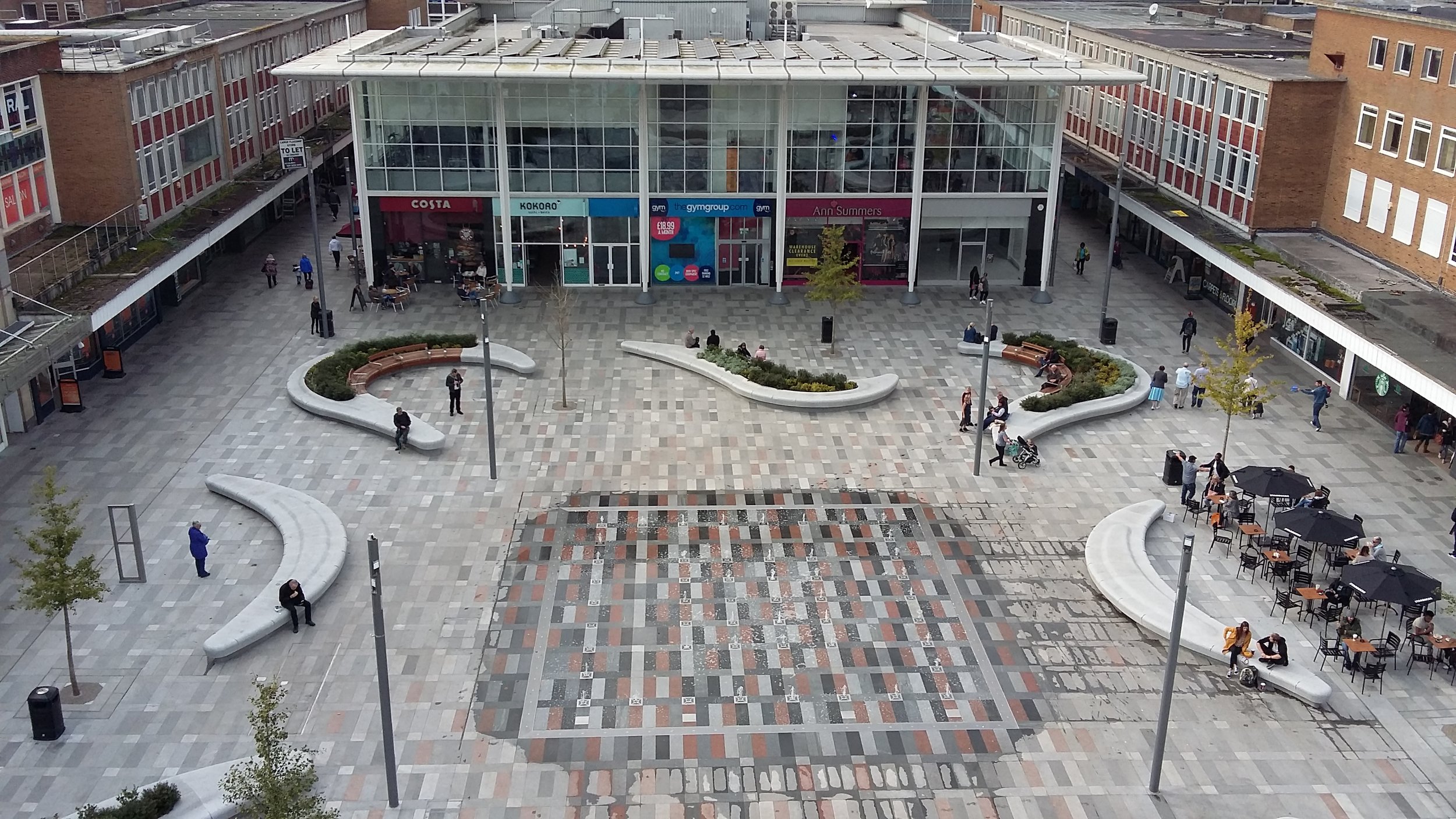This aerial photograph captures an expansive courtyard bordered by buildings, taken from approximately 20 to 30 feet above at a slight angle. The courtyard floor features a striking tile pattern; the central area is composed of darker, richer shades of dark gray, black, and dark red tiles, while the surrounding tiles are lighter neutral colors. Curved stone benches are strategically placed in the courtyard, with the top three benches adorned with small plants and bushes in the center. People are seen sitting on these benches as well. Toward the center at the top of the image, there is a larger building front featuring five different storefronts with various colored banners: "Costa" in white on maroon, "KOHDAD" in black on teal, an unreadable white-on-blue sign, "Ann Summers" in gold on dark purple, and an unmarked gray banner on the far right. Additionally, there are buildings on the left and right sides of the courtyard. On the right side, one restaurant features outdoor seating with tables, chairs, and umbrellas. A few people are visible walking around the courtyard, adding a lively atmosphere to the scene.